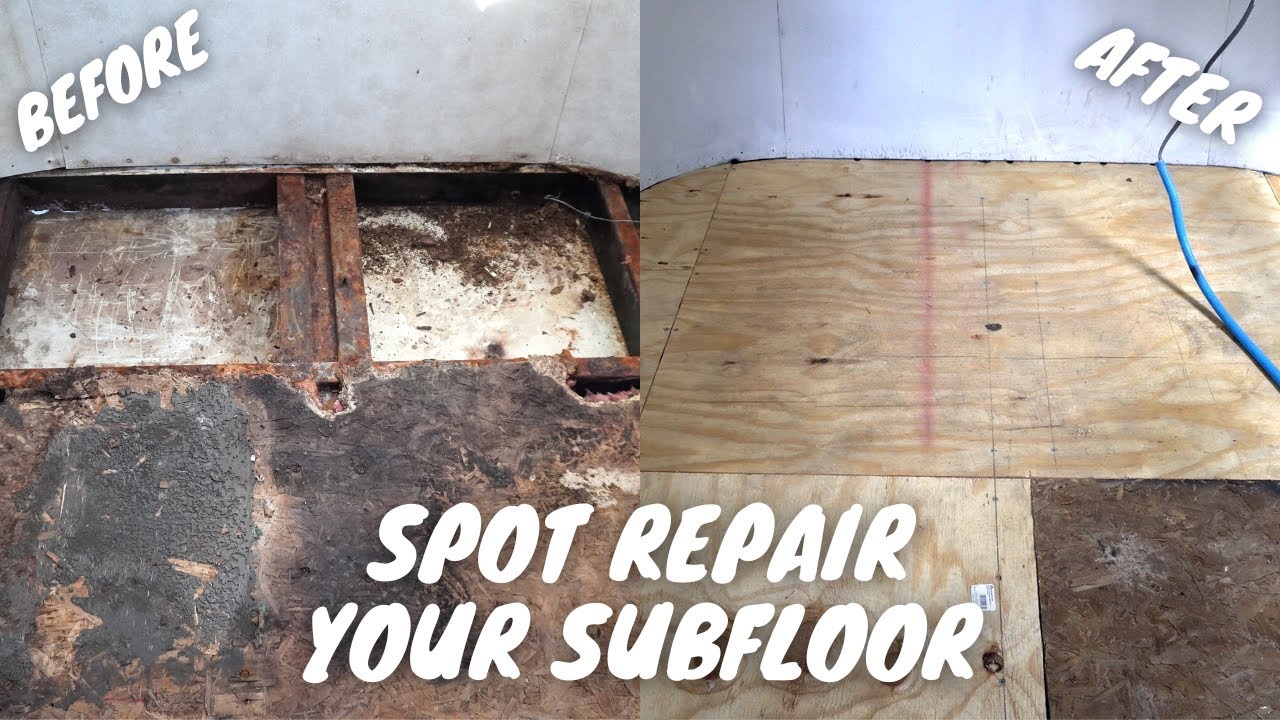The image showcases a dramatic before-and-after transformation of a subfloor repair project, likely posted by a subfloor repair business. The left side of the image, labeled "BEFORE" in white letters, displays a severely damaged, dirty, and rotted floor riddled with grime, mold, and cobwebs. This would be a frightful sight for any homeowner. By stark contrast, the right side of the image, labeled "AFTER" in white letters, reveals a meticulously reconstructed subfloor made of clean, unfinished wood, completely free of debris and damage. Both sections of the image feature a caption at the bottom that reads, "SPOT REPAIR YOUR SUBFLOOR," reinforcing the service offered. Notably, the only additional element in the "AFTER" photo is a solitary blue wire, indicating some ongoing electrical work.